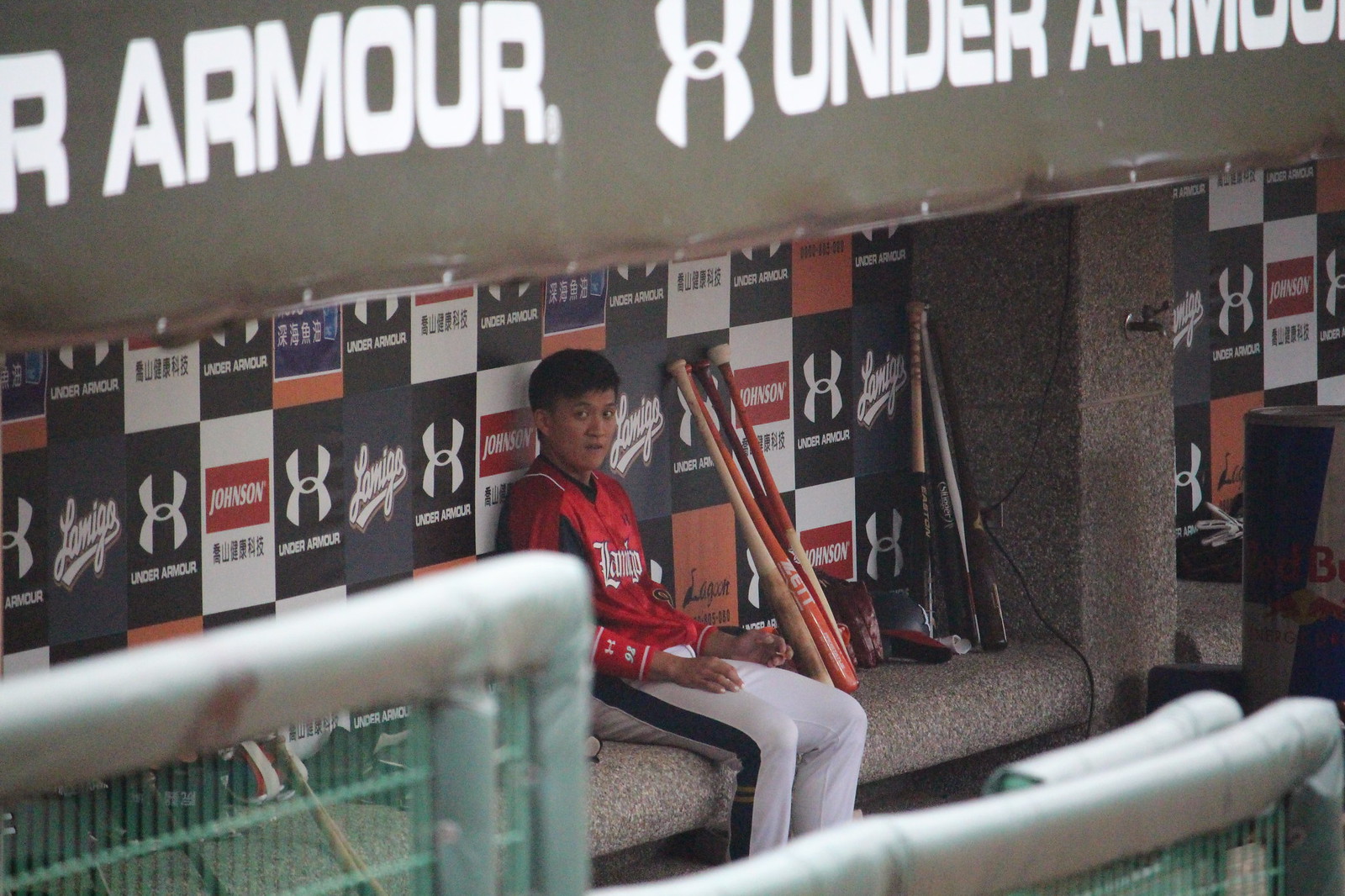A baseball player with short, dark black hair parted on the right sits alone on a bench in a baseball dugout, facing right but looking back towards the center. He wears a red jersey with white lettering, though the text is too small to read, and white pants featuring a black stripe down the side. The dugout's walls are adorned with various advertisements: a prominent black banner with white text for Under Armour, showcasing the distinctive logo of two U's (one upright, the other upside down), and a red square advertisement bearing the name Johnson, with additional text in a foreign language. The name Lamigo can also be seen among the logos, repeated in a tile format along the walls. Several baseball bats of different colors—red, brown, tan, orange, and black—lean against the wall, accompanied by gloves and hats scattered around. The dugout also features green fencing with grey padding near the front, partially blocking off the area but still providing a clear view of the solitary player amidst the backdrop of light green upper walls.